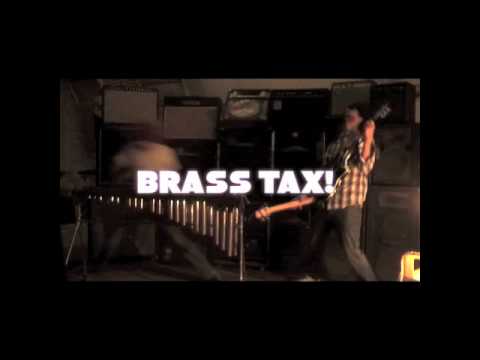In a dimly lit, indoor setting, a strikingly blurry and faded full-color photograph frames the scene of a chaotic yet joyous impromptu musical jam session. The centerpiece of the image is bold, white capitalized text reading "BRASS TACKS!" The poorly captured picture seems almost monochrome due to its low quality, making the outline of two young musicians barely discernible. On the right, a boy wearing a plaid shirt is engrossed in playing a guitar, another guitar hanging at his side. Nearby, another kid is hunched over a xylophone-like instrument, although completely out of focus as if caught moving when the photo was snapped. Stack amplifiers line the background, reinforcing the makeshift garage band vibe. The black border around the image suggests it might be either a poster or promotional material for a band named "Brass Tacks."